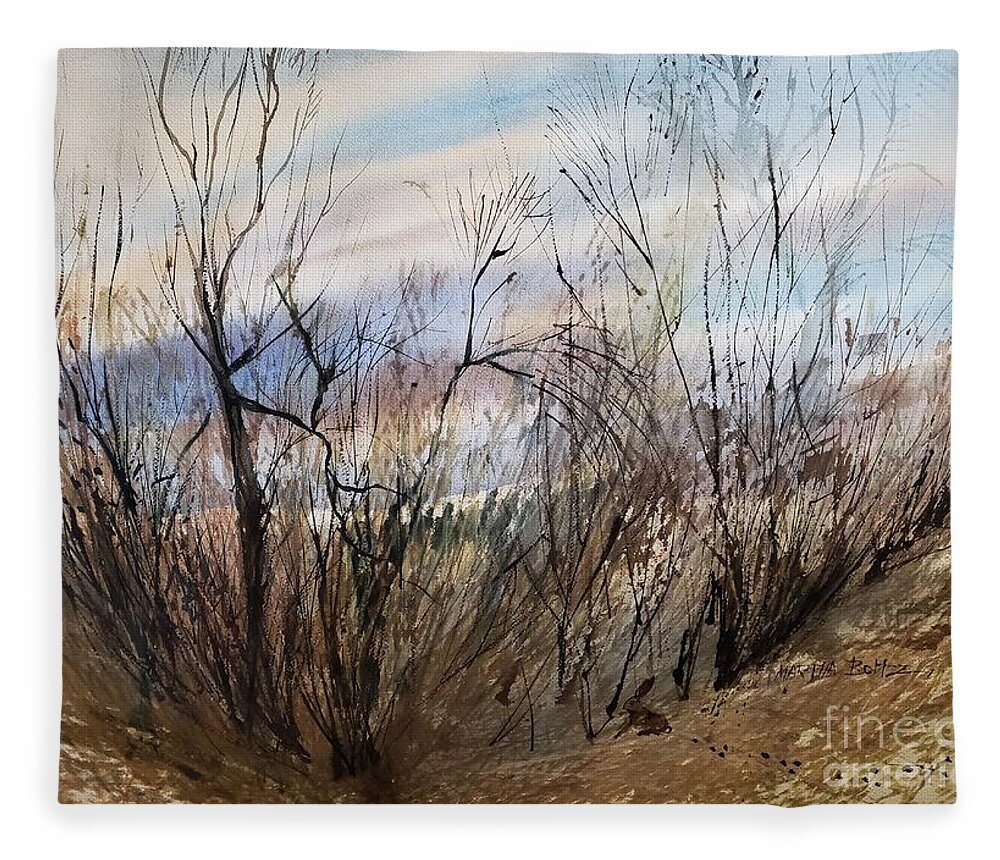The image is a detailed photograph of a hand-painted canvas art, prominently showcasing a winter prairie scene. The canvas is dominated by somber, neutral tones with subtle hints of color, featuring a thicket of thin, leafless black trees and shrubs, which stretch across the center of the composition. The dark branches, almost black, create a stark contrast against the muted ground, tinged with orange, and the lively yet subdued sky. The sky in the background melds through shades of blue, purplish, white, and a touch of yellow, with thin, streaky clouds enhancing the somber mood of the painting. Amidst the dense foliage near the bottom right-hand corner, blending almost imperceptibly with the surrounding dark branches, a small black bunny rabbit can be seen. The painting includes a watermark and possibly a signature in the lower right-hand corner, indicating it's a piece of fine art. The entire scene, with its coarse, branchy lines and melancholic ambiance, evokes a sense of stark beauty and desolation.